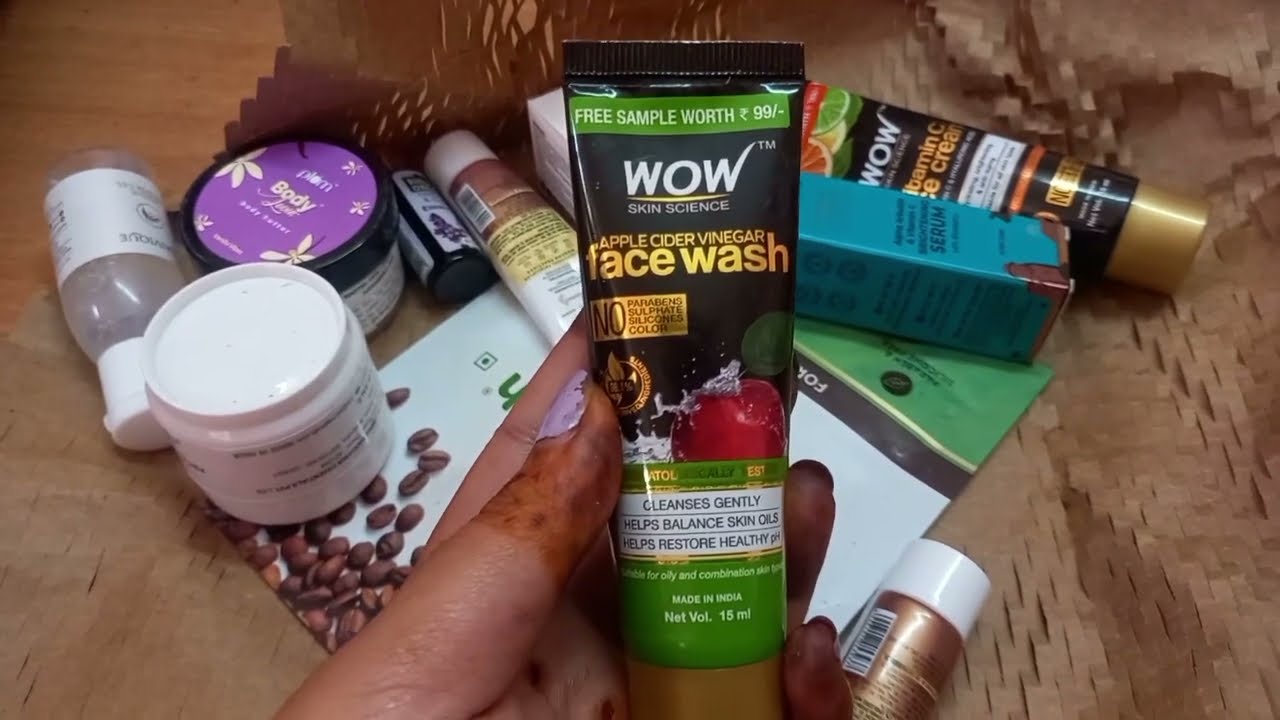In this image, a woman's left hand with light brown skin, blotched with henna-like stains on her fingertips and adorned with purple nail polish, is holding up a black and green tube of apple cider vinegar face wash by Wow Skin Science. The tube features white and gold lettering along with an image of an apple and is labeled as a free sample. The backdrop consists of brown packing paper or a tablecloth with a wicker-like appearance, on which various other beauty product samples, including canisters and tubes, are scattered. Among these, there are containers identified as vitamin C facial cream and possibly a facial serum.